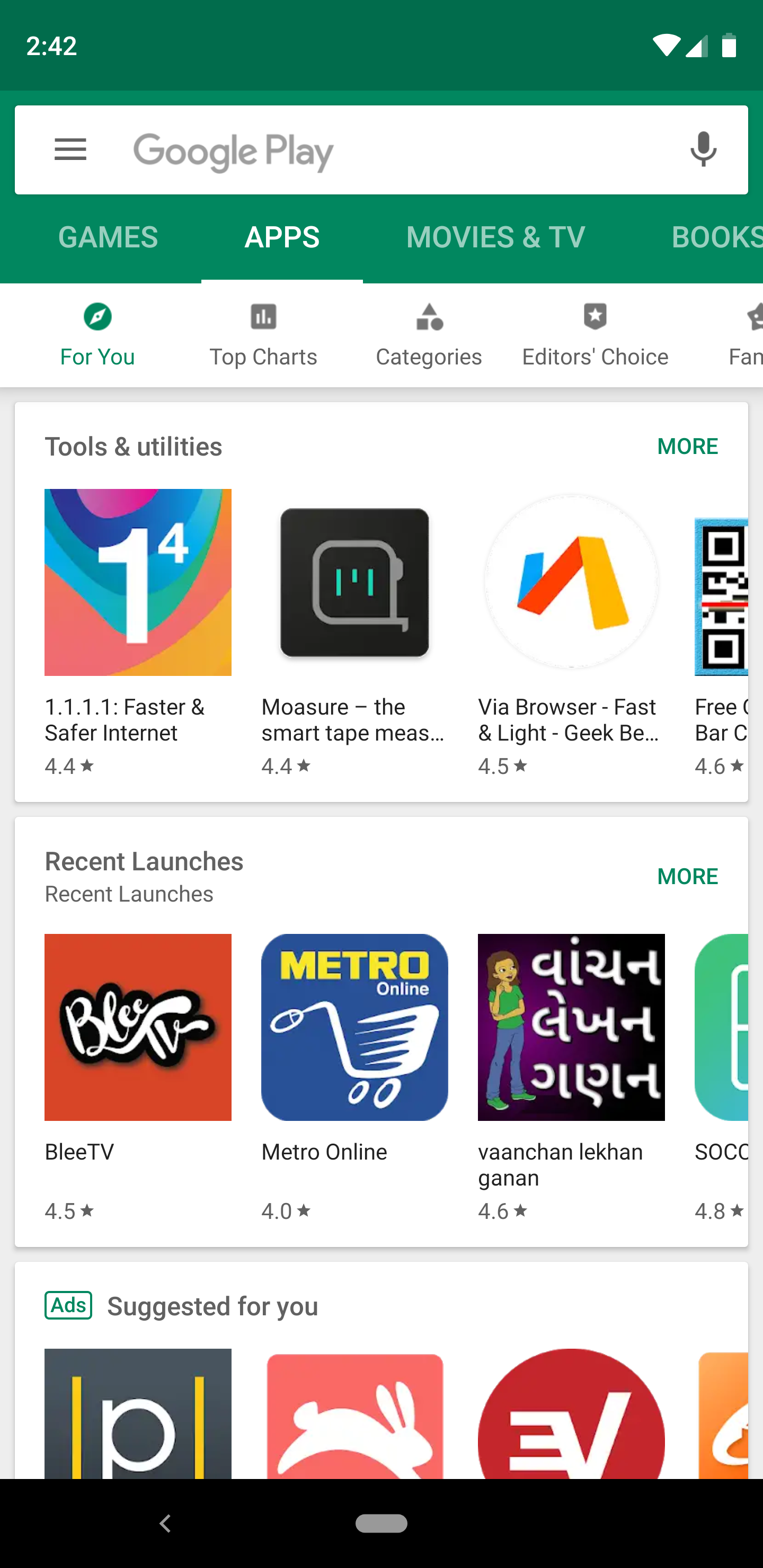**Screenshot of Google Play Store on a Mobile Device**

The screenshot captures a mobile device’s screen displaying the Google Play Store interface. The device shows the time as 2:42, connected to Wi-Fi with three-quarters signal strength, and a battery level between 80% and 90%. 

At the top, the Play Store features a green banner with a search box, a microphone for voice searches, and a menu button. The tabs available under the banner include Games, Apps, Movies & TV, and Books. The Apps tab is currently selected. Subcategories visible are For You, Top Charts, Categories, Editor's Choice, and Fan Favorites (the last option is cut off). Within these subcategories, "Top Charts" is highlighted.

Below the subcategory tabs, various app carousels are displayed. The first carousel titled "Tools and Utilities" includes the following apps:

1. **1.1.1.1 Faster & Safer Internet** - Features a rainbow-colored logo with the number 1 and has a rating of 4.4 stars.
2. **Moasure - The Smart Tape Measure** - Displays a black square with a ghost-like figure and holds a 4.4-star rating.
3. **VIA Browser - Fast & Light, Geek** - Has a circular logo in blue, red, and yellow with a reversed 'N', rated at 4.5 stars.
4. An app with a QR code icon, named "Free" (partially cut off).

Below the Tools and Utilities section, there is another carousel titled "Recent Launches," showcasing these apps:

1. **BLE TV** - Features a red box with vintage text, rated 4.5 stars.
2. **Metro Online** - Displays a blue box with a mouse-shaped shopping cart and the text "Metro" in yellow and "Online" in white, rated 4 stars.
3. **Vanchan Lekhan Ghanan** - Shows a purple and black box with a figure of a brown-skinned woman and foreign text, rated 4.6 stars.
4. An app with a green and blue icon reading "SOC" (partially cut off), rated 4.8 stars.

At the bottom, an ad carousel labeled "Suggested for You" appears, showcasing various partially visible ads including a gray box with a white 'P', a pink box with a white rabbit, a red circle with backwards 'VE', and an orange box with a white logo.